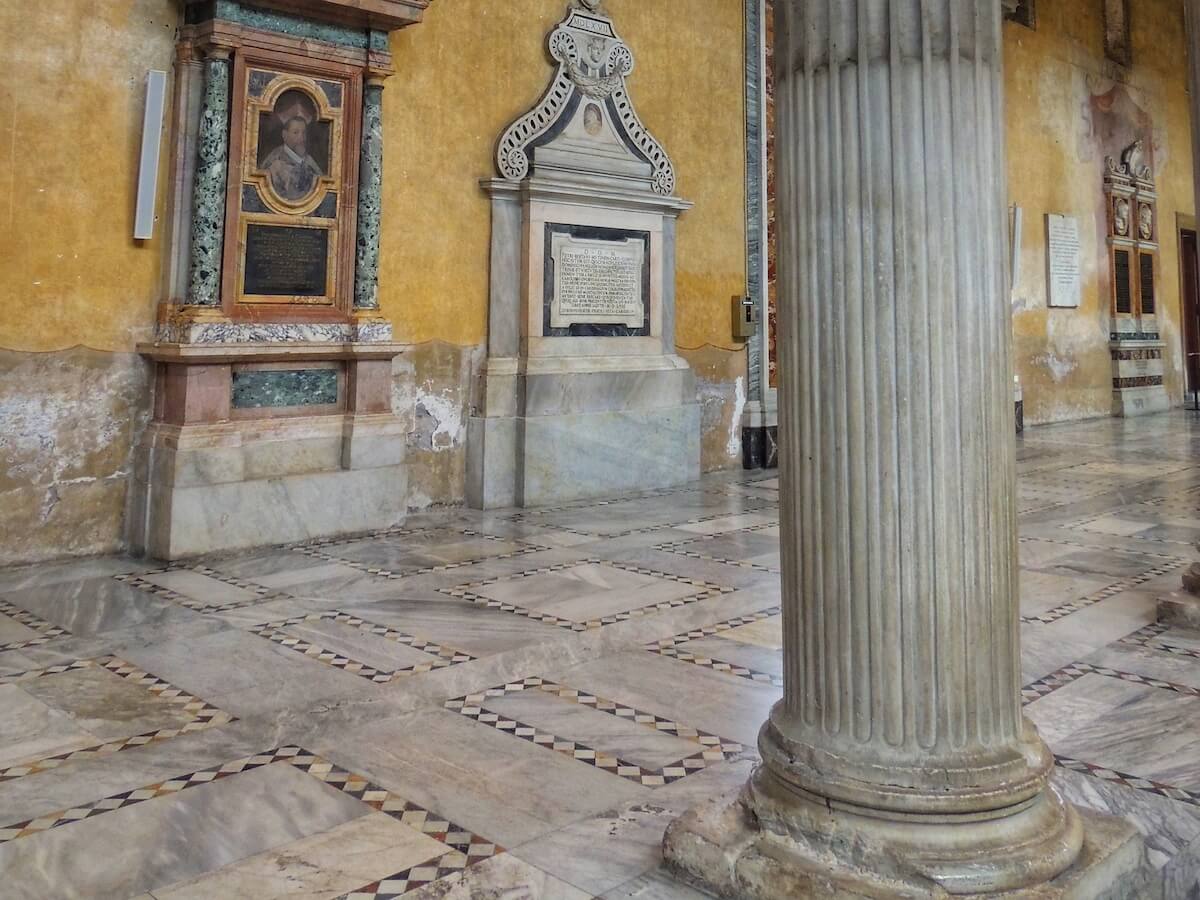The image captures the interior of a historic European church, with detailed and ornate features indicative of its religious significance and considerable age. The floor is crafted from polished marble tiles, arranged in rectangular and square mosaic patterns that reflect the surrounding architecture. Prominently in the foreground stands a large, weathered stone pillar, likely marble, with visible vertical lines and some erosion at its base. The walls, painted a distinct yellow, host a variety of artifacts, including a marble monument adorned with extensive but unreadable inscriptions. Another notable feature is an old painting of a man with a long beard wearing a bishop's hat and robe, framed in gold and flanked by green marble pillars. This painting, along with other religious figures displayed on the walls, hangs above a plaque with text that remains unclear. The scene is enhanced by the presence of a fluorescent light mounted on the wall, adding a mix of classical and modern elements to the sacred and historical ambiance of the site.